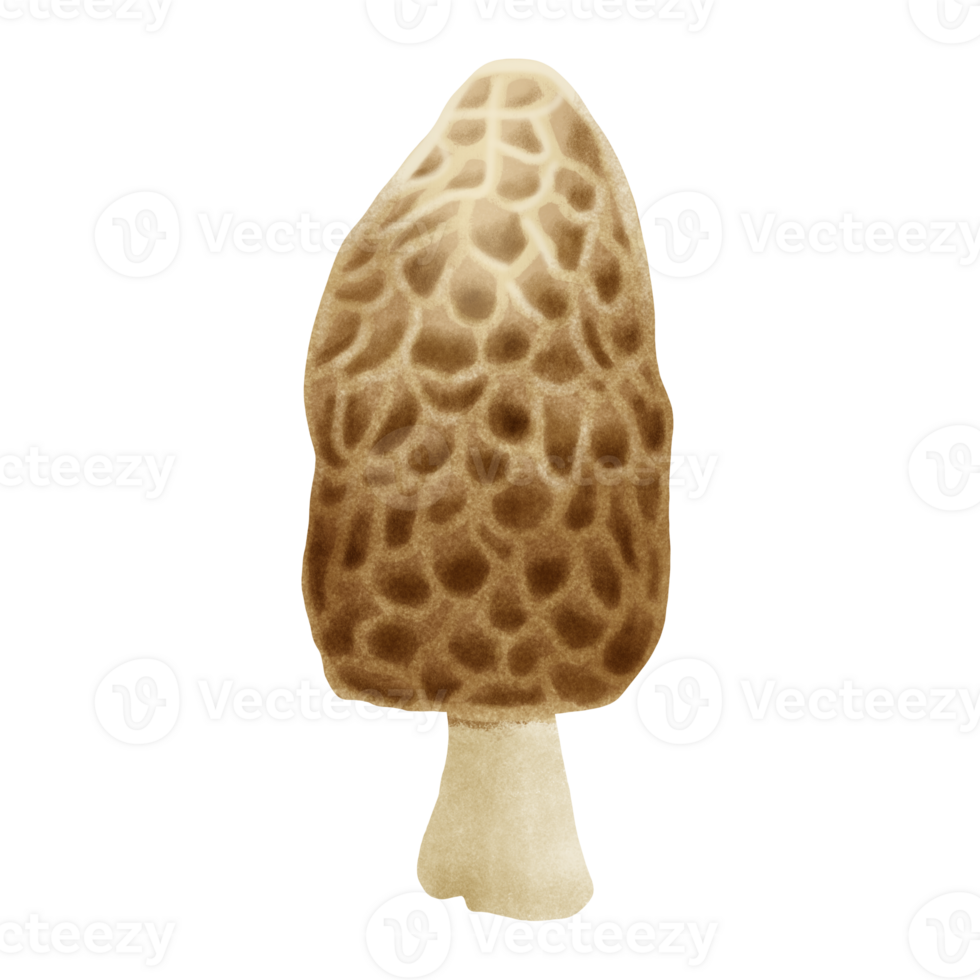The image showcases a highly detailed illustration of a morel mushroom, renowned for its luxury status and exquisite value. The mushroom features a distinct white stem resembling the leg of a typical mushroom, which transitions into a tall, almost closed, umbrella-like cap. The cap itself is light brown with darker brown interiors in its numerous, irregularly shaped holes. These holes create a spongy, honeycomb-like texture, akin to the chambers of a sponge. The mushroom appears as if it has a slightly pointy top and a relatively flat base, adding to its unique structure. Additionally, there's a faint watermark that reads "Vic TZ" with a V logo, subtly visible on the illustration.